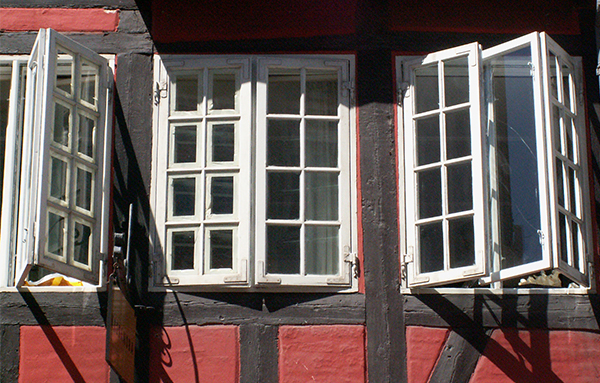The image depicts an old, large wooden structure that resembles a red and black barn-like house or possibly an old pub or business establishment. The building is constructed of red-colored wood with noticeable black wooden planks arranged both vertically and horizontally. prominently features three large, side-by-side windows with white frames. These windows are outfitted with grids of glass panels and are divided by wood beams. The windows open outward, with the side windows having hinges along the middle, which allow the panes to angle inward. Although in the photograph, two of the windows are distinctly open. There is also a sign on the building, though the text is not easily readable.